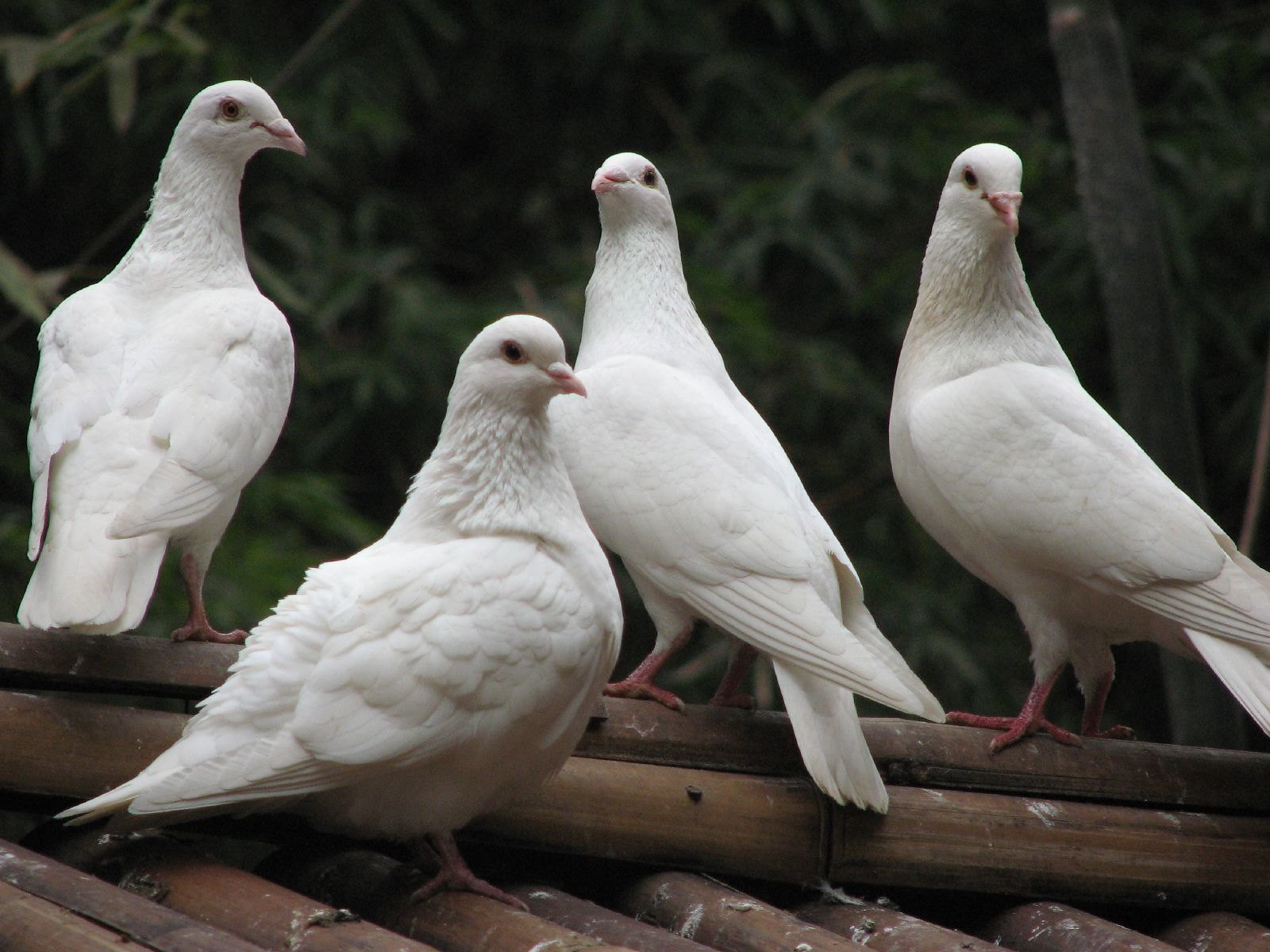This is a detailed photograph of four almost completely white pigeons perched on a structure that appears to be a wooden or bamboo roof with a slope. The wood forms a cross beam on which the pigeons are resting. Three of the pigeons are looking off to the right, while one is looking to the left. Their beaks vary slightly in color. Behind the pigeons, the background reveals shadowy green foliage, suggesting a backdrop of trees or shrubbery, with hints of bamboo possibly visible on the right side of the photograph. The pigeons are facing towards the camera but not directly looking at it, creating an image where they are central yet not the focal point.